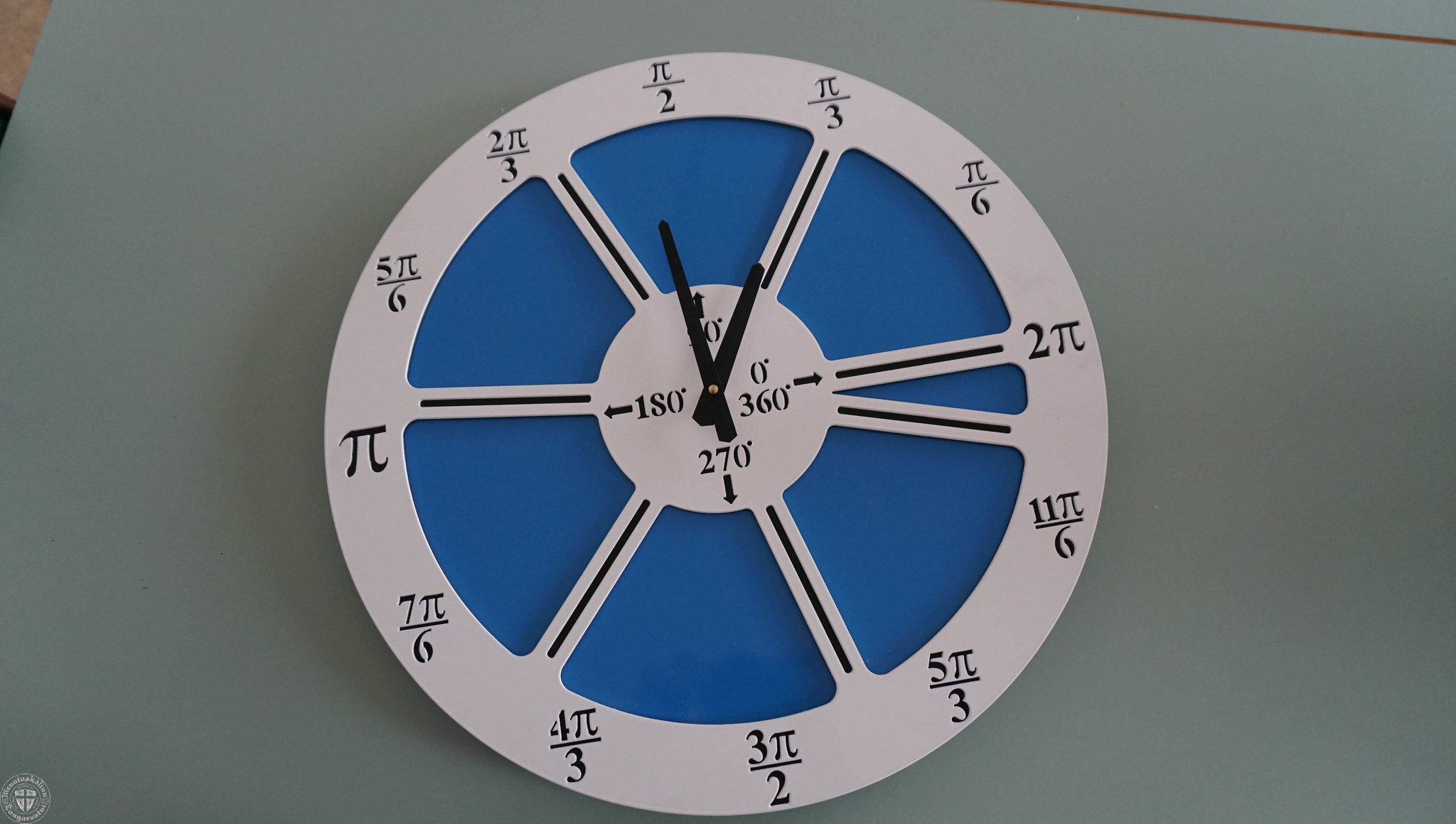This image features a unique clock displaying a non-traditional arrangement of angles in radians instead of standard numeric hour markers. Starting from the top and moving clockwise, the positions are labeled as follows: π/2 (pi divided by 2) at the top, π/3 (pi divided by 3) at the first position clockwise, π/6 (pi divided by 6) next, followed by 2π (2 pi), 11π/6 (11 pi divided by 6), 5π/3 (5 pi divided by 3), 3π/2 (3 pi divided by 2), 4π/3 (4 pi divided by 3), 7π/6 (7 pi divided by 6), 5π/6 (5 pi divided by 6), 2π/3 (2 pi divided by 3), and finally π/2 (pi divided by 2) again. The arrangement doesn't follow the typical numerical progression of a standard clock, instead using mathematical constants and radian measures to mark each hour. This unconventional design makes it a fascinating piece, merging the concepts of time and mathematics in a visually intriguing manner.